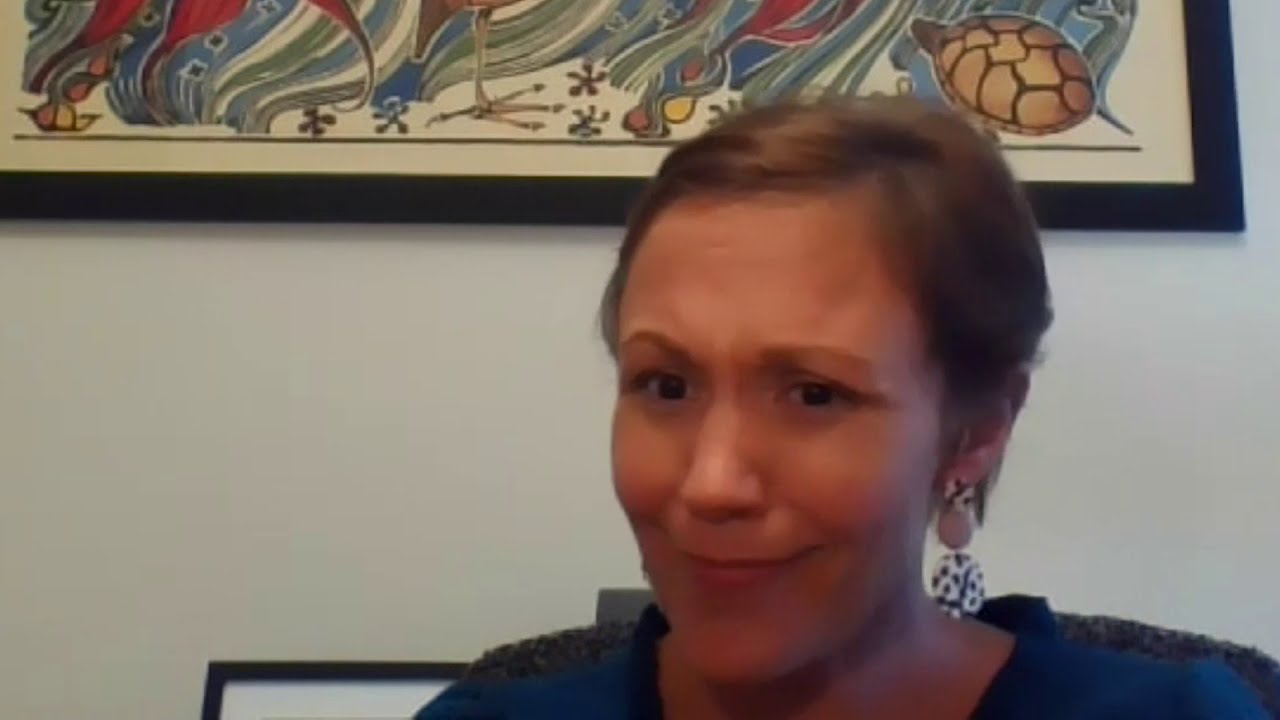In this detailed color photograph, a woman with short brown hair stands slightly off-center to the right against a stark white wall. She wears a blue shirt, and only her shoulder and above are visible. The woman, who appears embarrassed or concerned, has a neutral expression with her mouth closed and slightly lifted as if scowling. Her eyebrows are furrowed as she gazes downward and slightly to the left. She sports distinctive white earrings adorned with a black dot pattern. Behind her, there is a black-framed artwork almost occupying the top portion of the image. The artwork features animal drawings, notably a turtle in the bottom right corner. Additionally, the back of a gray upholstered chair is faintly visible behind her.